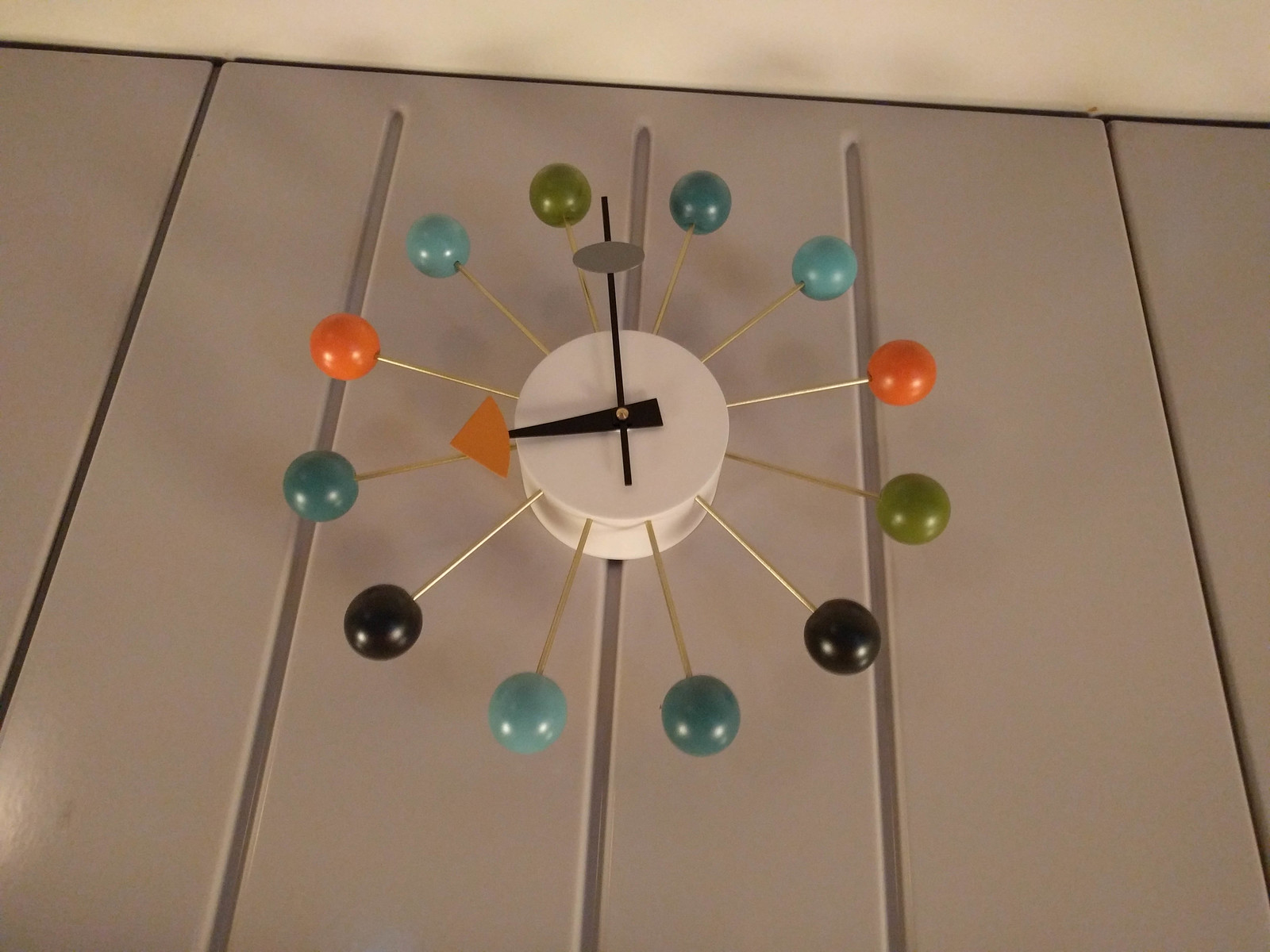In this horizontally elongated, rectangular image with a lower resolution that gives it a vintage feel, we see a photograph depicting a classic Art Deco-style wall clock. The clock is mounted against a light-paneled wall with a cream-colored ceiling above. The clock's centerpiece is a white circular face featuring two dark-colored hands with geometric accents — the hour hand adorned with an orange triangle and the minute hand ending with a gray oval. Extending outwards, reminiscent of wheel spokes, are numerous rods each capped with a circular bead-like embellishment. The embellishments are a vibrant array of colors, including orange, light blue, avocado green, and black, enhancing the clock’s retro aesthetic.